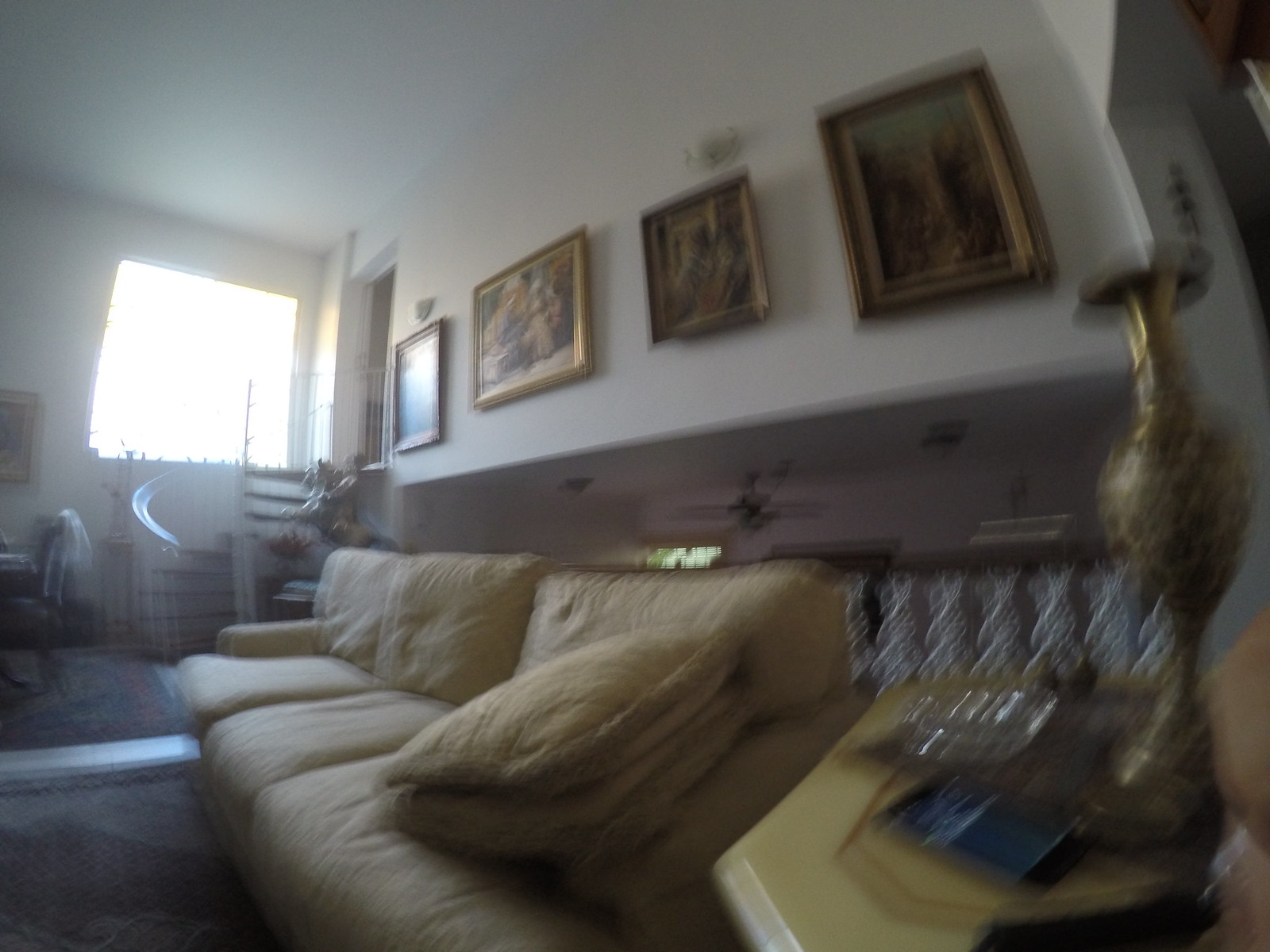In this slightly blurry, first-person perspective photo taken at waist height, a cozy living room or den area of a home is depicted. At the foreground on the right, an aged, beige-yellow end table holds an ornate golden vase, a glass dish, and a partially obscured blurry item, likely a phone. A long, mustard-yellow couch with several cushions takes up the left side, seating around six to eight people. Behind the couch, a unique banister features glass balusters that are thicker at the base and taper towards the top. A set of staircases is partially visible on the left, ascending towards a doorway. Additionally, the living room is bathed in natural sunlight filtering through a window on the far left. Above the banister on the white upper wall, four various-sized, gold-framed artworks are displayed. A slight gap between the railing and the upper wall reveals part of the lower level or entranceway ceiling, hinting at the multi-level layout of the home.